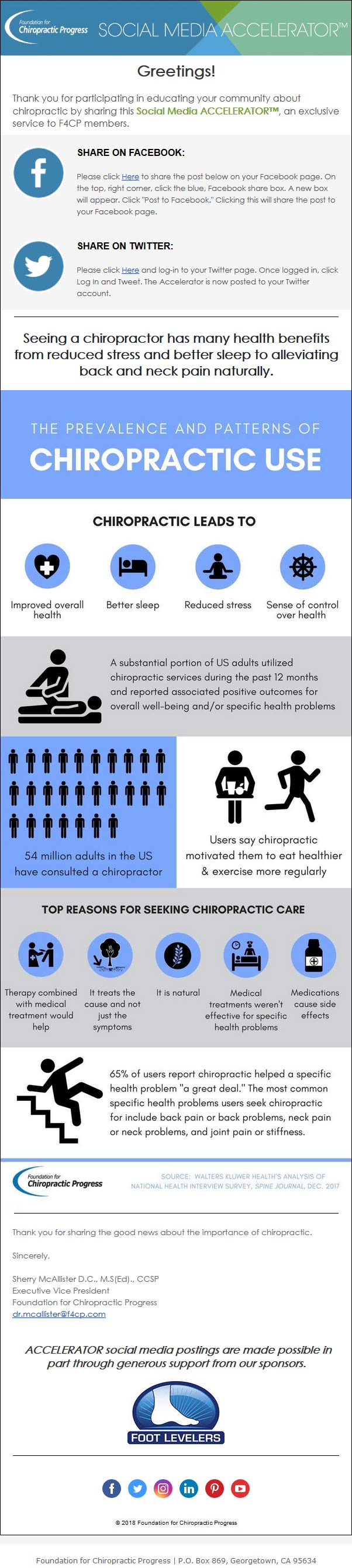The image is a long informational poster or banner designed for chiropractic use, prominently displaying the title "Social Media Accelerator" in green tones at the top. It serves to educate the community about chiropractic through social media, with a primary white background accented by blue and black fonts, and gray bars at the top. The poster opens with a greeting and invites participants to share the content on social media platforms such as Facebook, Twitter, Instagram, LinkedIn, YouTube, and Google, indicated by their respective icons at the bottom.

Central to the poster is a large blue bar with white text reading "Prevalence and Patterns of Chiropractic Use." Below this, another white section provides benefits of seeking chiropractic care, including improved mental health, better sleep, and reduced stress. An illustration of a chiropractor with a patient and additional diagrams, though present, contain text that is too small to read. Despite the small font size affecting readability, the poster effectively uses blue circles, diagrams, and other visual elements to convey its message.